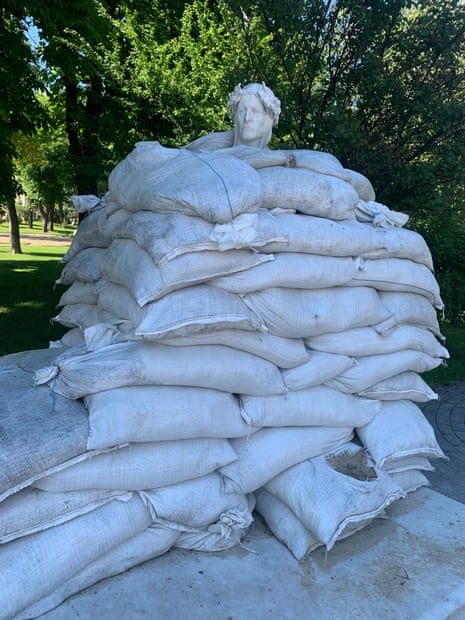The image depicts a marble sculpture of a classical-style figure, presumably a man, adorned with a laurel wreath on his head. This statue is set in an outdoor, shaded park area filled with greenery and large trees, creating a dappled light effect as sunlight filters through the leaves. The statue is partially obscured by a triangular formation of white sandbags that are piled up to the figure's throat. These sandbags, with at least one torn open revealing sand or dirt inside, seem to be protecting the statue, possibly from flooding. The base of the statue is made of stone or marble, accentuating the classical aesthetic. The background features the lush canopy of a large tree and additional trees, contributing to the serene and secluded atmosphere of the park on what appears to be a bright, sunny day.